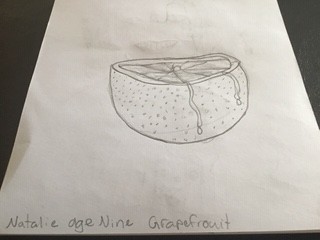This photograph captures a child's pencil drawing on a smudgy white piece of paper, showcasing a detailed sketch of a grapefruit with its top cut off. Positioned centrally on the page, the grapefruit appears in a 3D style, complete with visible segments, outer rind texture, and drips of juice running down its sides. At the bottom of the drawing, written in pencil, are the words "Natalie, age nine, grapefruit," with "grapefruit" misspelled as "grapefrOuit." An additional, intriguing feature is the faint impression of a mouth and teeth over the left side of the grapefruit, likely a transfer from another sheet. Visible in the background are the black edges of the desk or table the paper is placed on, adding context to the artwork's presentation.